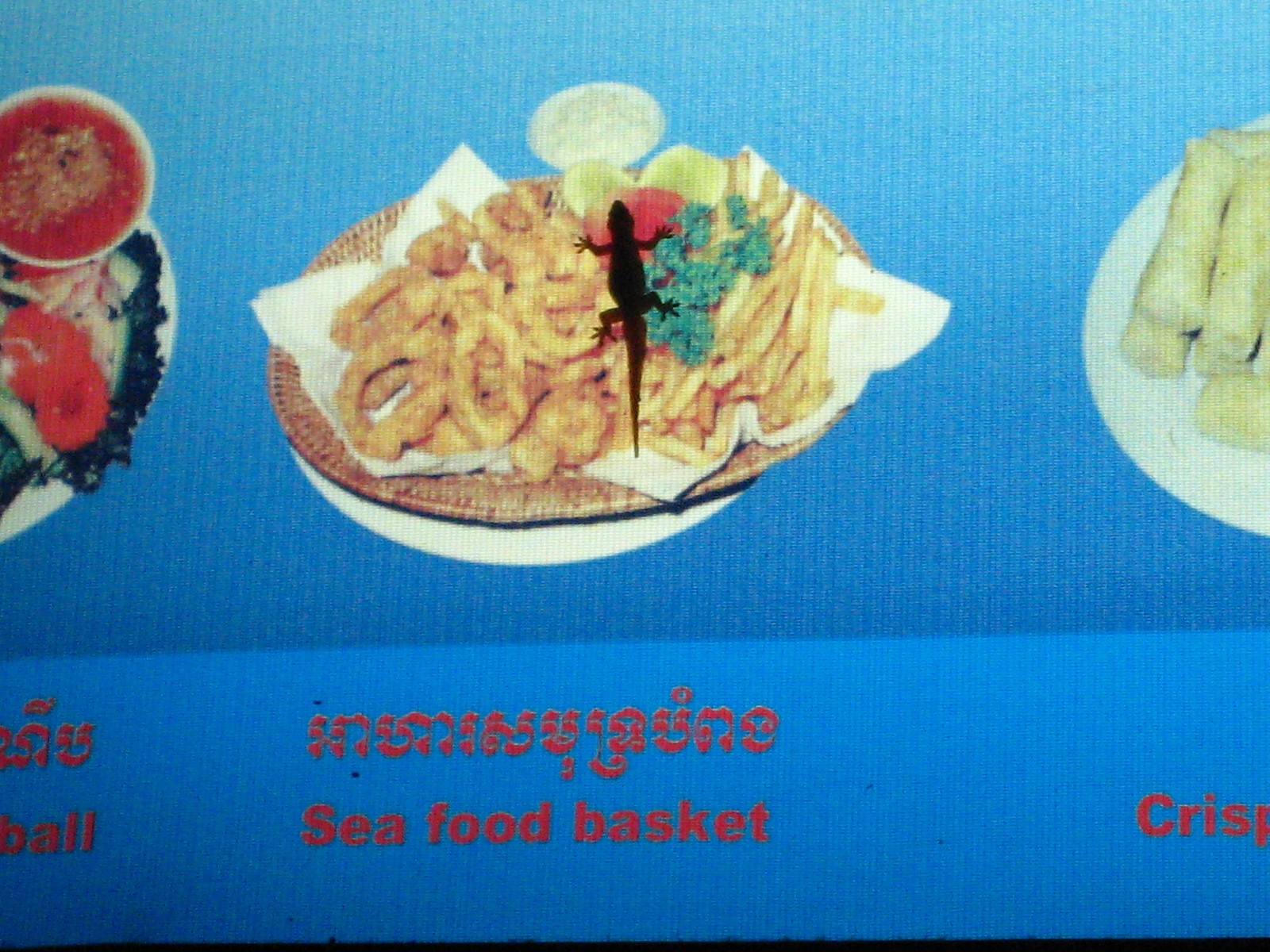The image depicts a section of what appears to be a menu, featuring various food items. The background is predominantly blue, with a darker, digital screen-like upper part and a lighter blue lower part. The text on the menu includes Thai characters and English translations.

At the center of the image is a detailed photo of a seafood basket, showcasing calamari, a garnish, lemon wedges, and French fries, all neatly arranged on a napkin within a basket. Above this central image, there is a small gecko or lizard resting on the screen, adding an unusual touch to the scene.

To the right of the seafood basket, another image captures a plate of spring rolls resting on a crisp, white surface. Although partially obscured, the text beneath it reads "spring rolls."

To the left of the central seafood basket image, there is an incomplete visual of what seems to be a dish labeled "ball" underneath Thai characters. This image, though partially cut off, reveals a red sauce or soup, accompanied by garnishes and vegetables.